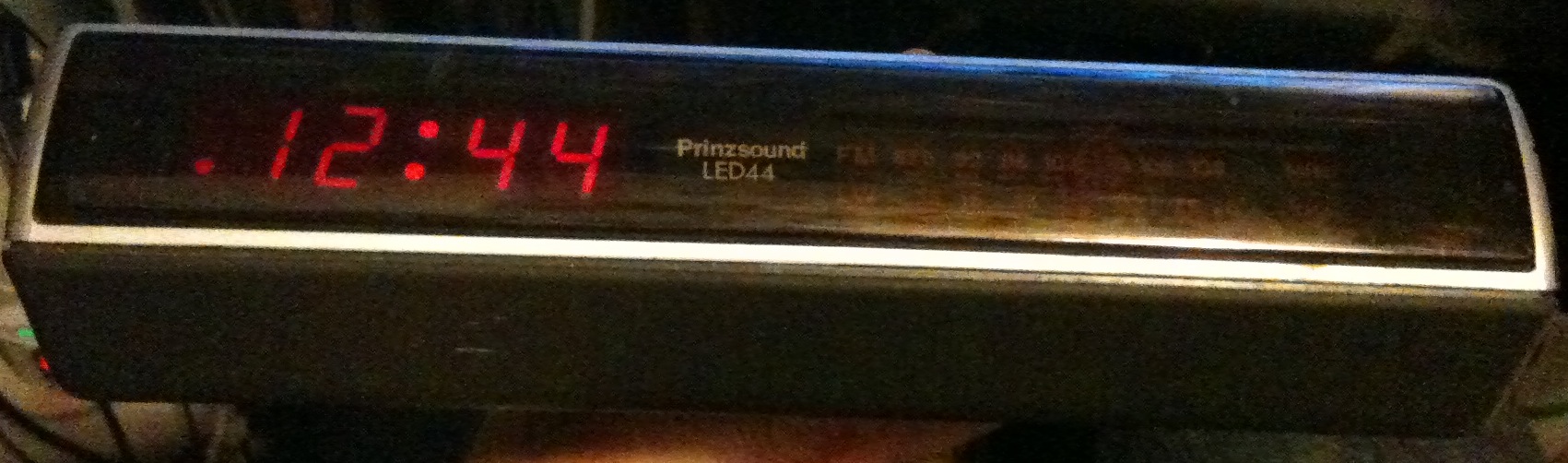The photo is a vertically-oriented, long and narrow image featuring a vintage alarm clock. This clock, boxy in design, gives off an older, somewhat worn yet functional appearance. The display reads "12:44" in classic red LED digits, with "Prince Sound LED 44" adjacent to the time. The clock itself is predominantly black with a touch of silver trim. The photo is taken from a slightly elevated perspective, revealing some details of the clock's possible radio function, although the FM/AM display is somewhat blurred. The background of the image is out of focus and cropped tightly around the clock.